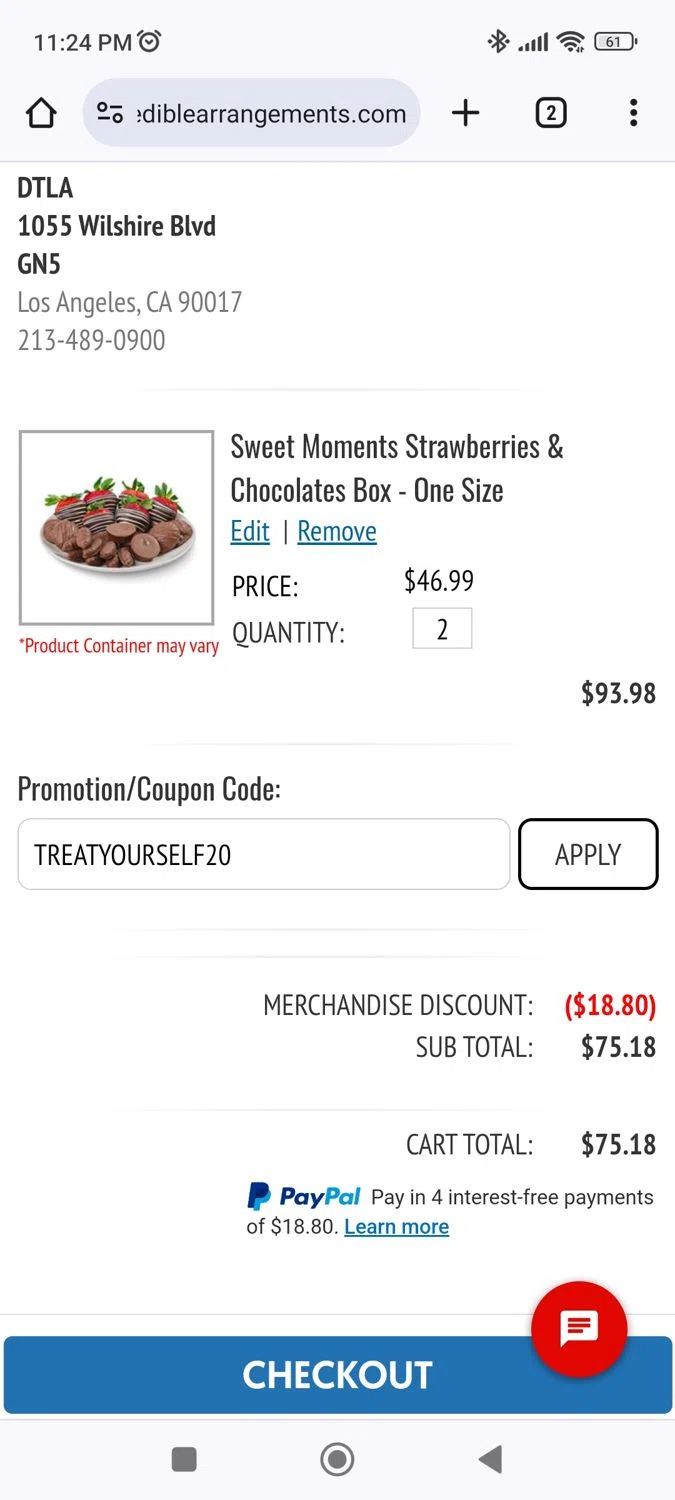The screenshot features an interface set against a clean white background. The header at the top is light gray, displaying dark black text. On the upper left corner, the time is shown as 11:24 PM with an alarm clock icon adjacent to it. Moving further right, the status icons indicate Bluetooth being on, full reception with all five bars lit, Wi-Fi connection active, and the battery status.

Below the header is a search bar and an address bar displaying "ediblearrangements.com." The main section below these bars shows the first item listed. The product name is "Sweet Moments Strawberries and Chocolates Box, one size." Options to edit or remove the item are available in blue text beneath the product name. The price is listed as $46.99, with a quantity of 2 specified. 

A color photo of the product is displayed to the left, highlighting a variety of chocolates in front of the platter and chocolate-dipped strawberries with their green tops intact positioned at the rear. The total price for the two items amounts to $93.98. Underneath the product listing, there is a box for entering a promotion coupon code.